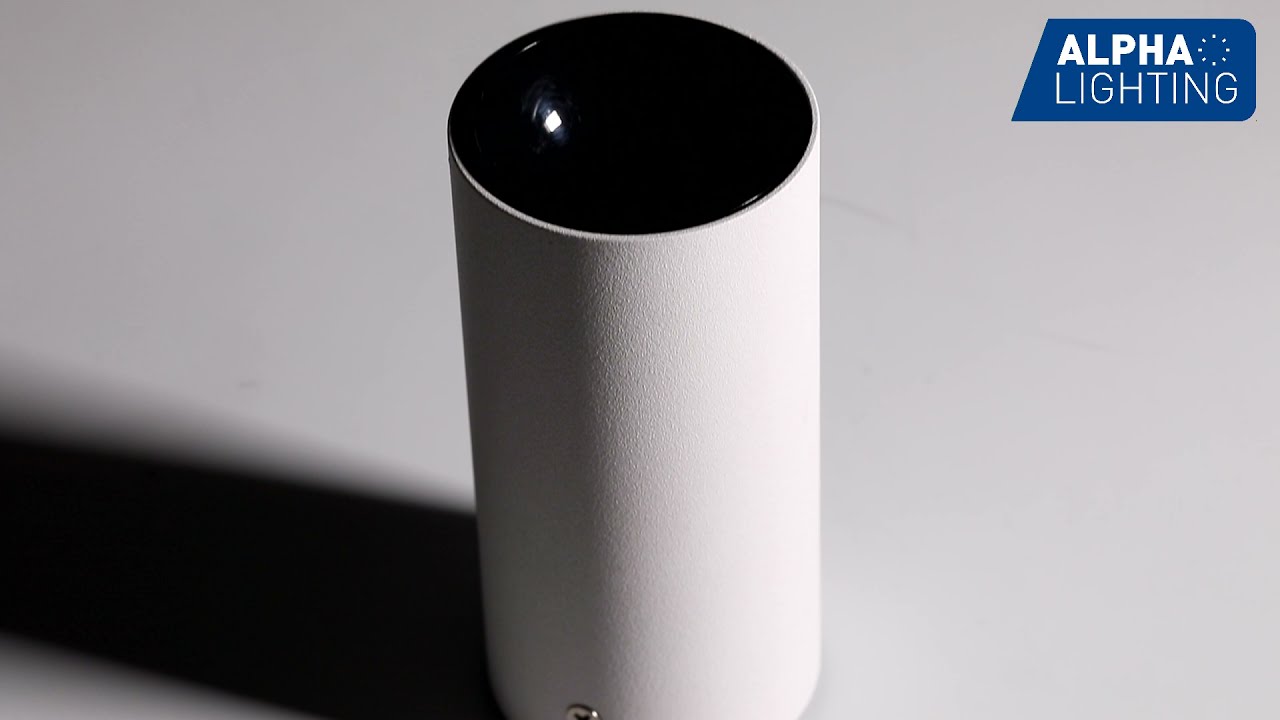This image depicts a sleek, cylindrical, white lamp with a black top, emitting a slender white light from its top. The lamp’s modern design is highlighted against a clean, white background with the lamp casting a noticeable shadow to the left. The top right corner of the image features a navy blue, slanted rectangular banner with the bolded, white text "Alpha Lighting" accompanied by a small white dotted circle next to the 'a' in "Alpha." The image, likely an advertisement or a product shot, isn't professionally framed as part of the lamp's base is cut off, and only the colors white, black, gray, and blue are present. The overall impression is one of a contemporary lighting device, blending functionality and minimalist aesthetics.